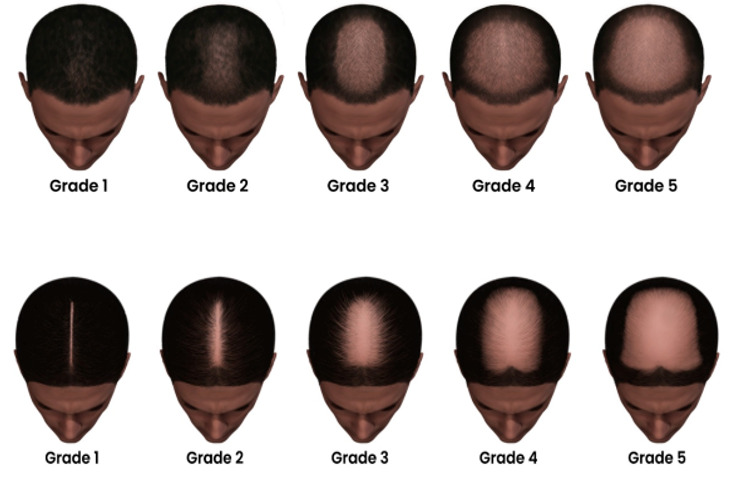The image showcases a comparative study of balding patterns in men, categorized into five distinct grades, numbered from one to five. The image is divided into two rows, with the top row depicting varying degrees of balding in African-American men, and the bottom row illustrating the same in Caucasian men. In both rows, each stage of balding becomes progressively more severe. At grade one, there are minimal signs of balding, mostly noticeable at the crown or the center part of the head. By grade two, the bald area has notably expanded. By grade three, a significant bald patch is visible, and at grade four, a substantial portion of the scalp is exposed. Finally, at grade five, the entire top of the head is bald. This detailed progression visually emphasizes the different patterns and severities of hair loss that men can experience, offering a clear comparative view across different ethnicities.